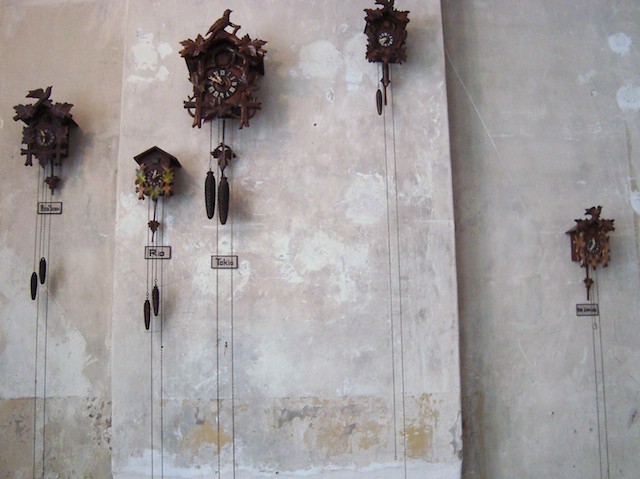This image captures a variety of brown cuckoo clocks meticulously arranged on a cement wall that features both smooth gray and tan sections with occasional white splotches. The wall is divided into three sections: on the far left, a single ornate cuckoo clock with a carved bird on top and a nameplate beneath it. The middle section is raised and hosts three more clocks. The first clock in this middle section is small, adorned with colorful birds on the front and a nameplate below. The second is the largest, boasting an intricate wooden bird on top, giant chimes hanging down, and a nameplate. The third clock in this central section is medium-sized and has a bird on top but lacks a nameplate, featuring just one chime. The far-right section holds the final, very small cuckoo clock which also has a bird atop it, colorful adornments on the front, no chimes, and a nameplate beneath. All clocks exhibit leaf patterns and pulleys, and their clock faces are black with white hands and numerals. The bottom of the wall shows some yellowing, adding an additional layer of detail to the backdrop.